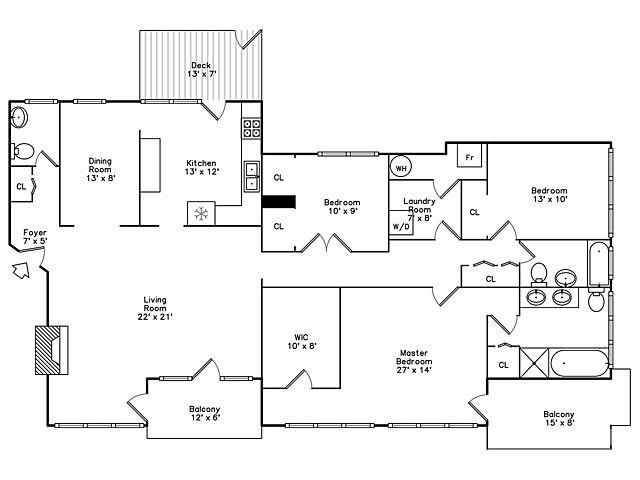This detailed black-and-white architectural drawing represents a sprawling one-story house plan. The home is divided into two main wings: the right wing and the left wing. 

The right wing includes three spacious bedrooms, each furnished with closets. It also houses a laundry room for convenience. The master bedroom is particularly feature-rich, with an en-suite bathroom. Additionally, a communal bathroom is located at the end of the hallway for shared use. Adjacent to this hallway is a 15'6" balcony, perfect for enjoying outdoor relaxation.

In the left wing of the house, designed in a semi-T shape, lies the primary living area. This section features a sizable living room measuring 21' by 20', a dining room, and a 13' by 12' kitchen fully equipped with all necessary appliances and fixtures. It also includes a bathroom for guest use. Complementing the living space are two outdoor areas: a deck on one side and another balcony on the opposite side, both offering additional options for leisure. The main entrance of the house opens into a 7' by 5' foyer, leading to the various parts of the home. 

The drawing meticulously details room dimensions, doors, and placements of fixtures like bathtubs, sinks, and toilets, providing a comprehensive view of the house layout.